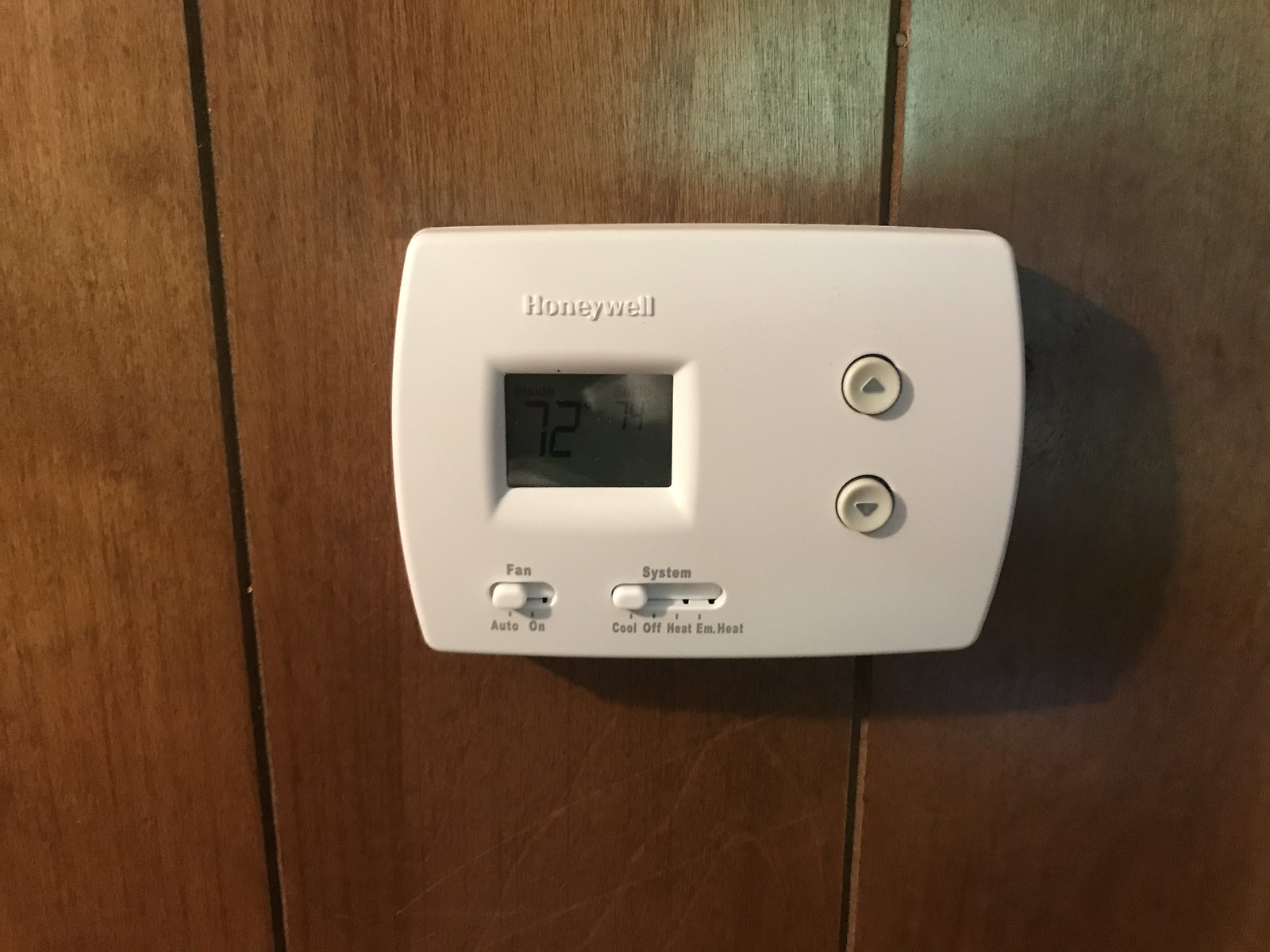This close-up photograph captures a thermostat unit mounted on an old-style wood-paneled wall. The wall features grooves between each panel and has visible wood grain ridges. The thermostat, a white plastic Honeywell unit, is horizontally oriented and spans across two wood panels. 

The Honeywell logo appears in raised font above the unit’s digital display, which shows the temperature set to 72 degrees in black font against a green background. Below the display are two sliding buttons. The left button is labeled "Fan" and has two settings: "Auto" and "On," both in light gray font. The right button is labeled "System" with settings listed as "Cool," "Off," "Heat," and "Exchange Heat," currently set to "Cool." On the right side of the thermostat are two circular buttons with gray arrows indicating up and down adjustments, respectively. 

The photograph provides a detailed view of the thermostat, highlighting both the device's interface and the textured wooden surface of the wall it is mounted on.